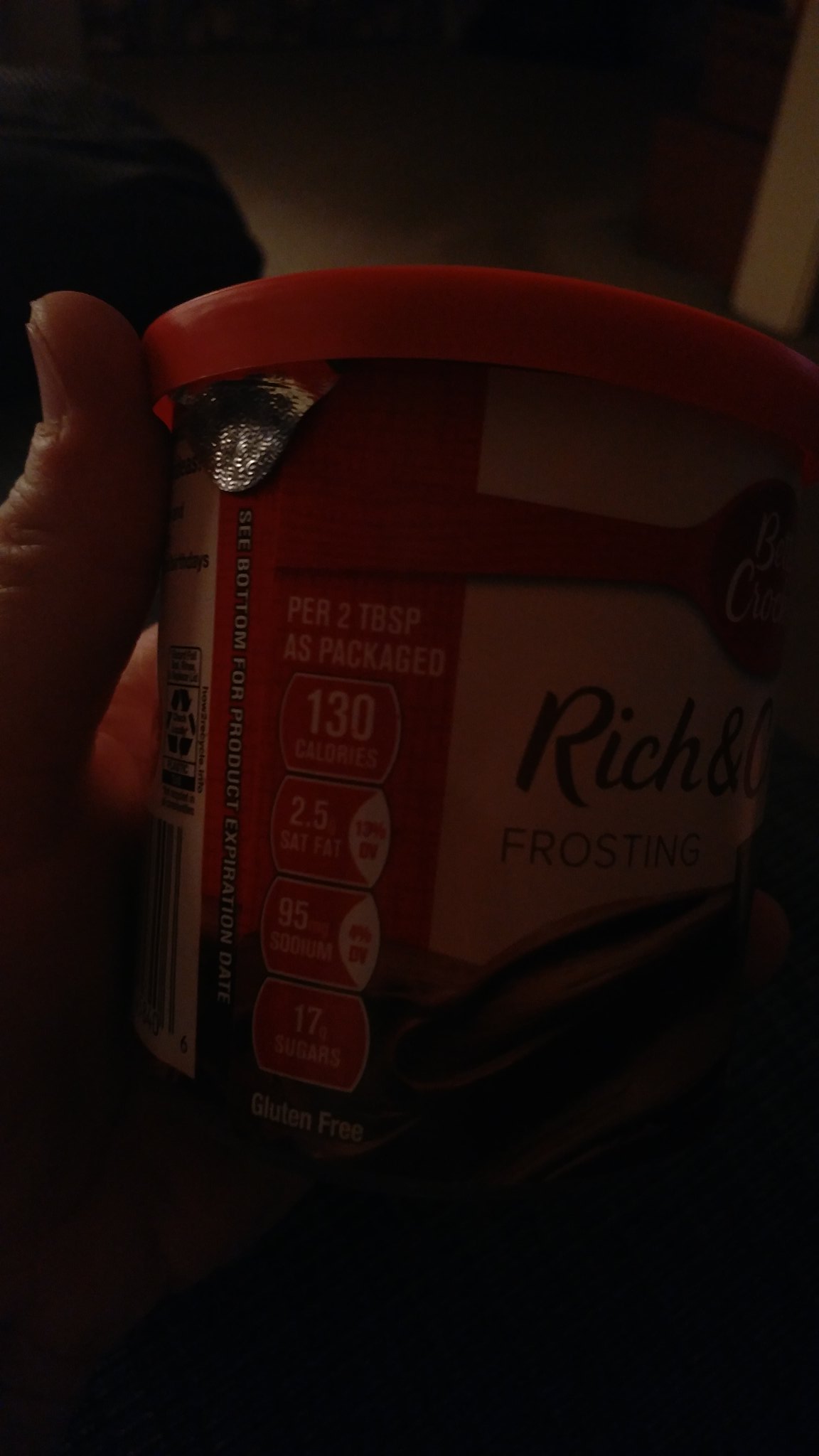In this image, a person is holding up a tub of a product, partially obscured by shadows. The scene is quite dark, making it difficult to discern the exact colors clearly. However, the lid of the tub is distinctly red. Positioned at the top left corner of the image, the person's thumb can be seen pressing against the side of the tub. The label on the product is partially visible and contains nutritional information. It reads "per tbsp," below which it states "as packaged," and further down it indicates that the product contains "130 calories." The details of the product label and the dark lighting give the image a mysterious and somewhat obscure appearance.